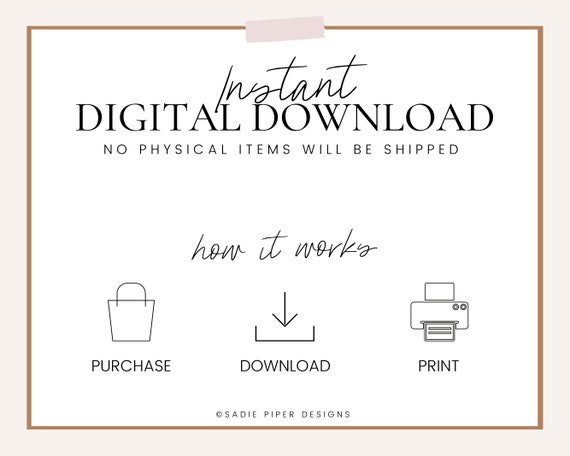This image is a detailed, digitally-generated advertisement featuring a step-by-step guide for an "Instant Digital Download." It is presented in landscape orientation and framed with a series of borders. The outermost border is a tan or beige color, about half an inch thick. Within this border is a thinner, approximately 3/16th inch dark brown or taupe border. The innermost section has a creamy white background.

At the top center of the image, a piece of tape is depicted, resembling a hand-drawn or computer-generated frayed edge, pastel in color—likely pale rose or mauve. Below this, in cursive script, the word "INSTANT" is prominently displayed. 

Following that, in all capital letters and a serif font like Times New Roman, the phrase "DIGITAL DOWNLOAD" is written. Subtly beneath this, in a smaller sans-serif font, the text "NO PHYSICAL ITEMS WILL BE SHIPPED" provides additional clarification. 

The guide continues with "HOW IT WORKS" written elegantly in cursive, higher up in the middle of the image. Below this headline are three simple, black-outlined icons paired with corresponding text instructions:

1. On the left is an outline of a trapezoidal shopping bag labeled "PURCHASE."
2. In the center, an arrow points downward toward an open bracket symbolizing a download slot, accompanied by the text "DOWNLOAD."
3. On the right, a basic printer outline with a sheet coming out is labeled "PRINT."

At the bottom of the image, the phrase "COPYRIGHT SADIE PIPER DESIGNS" marks the source of the content.